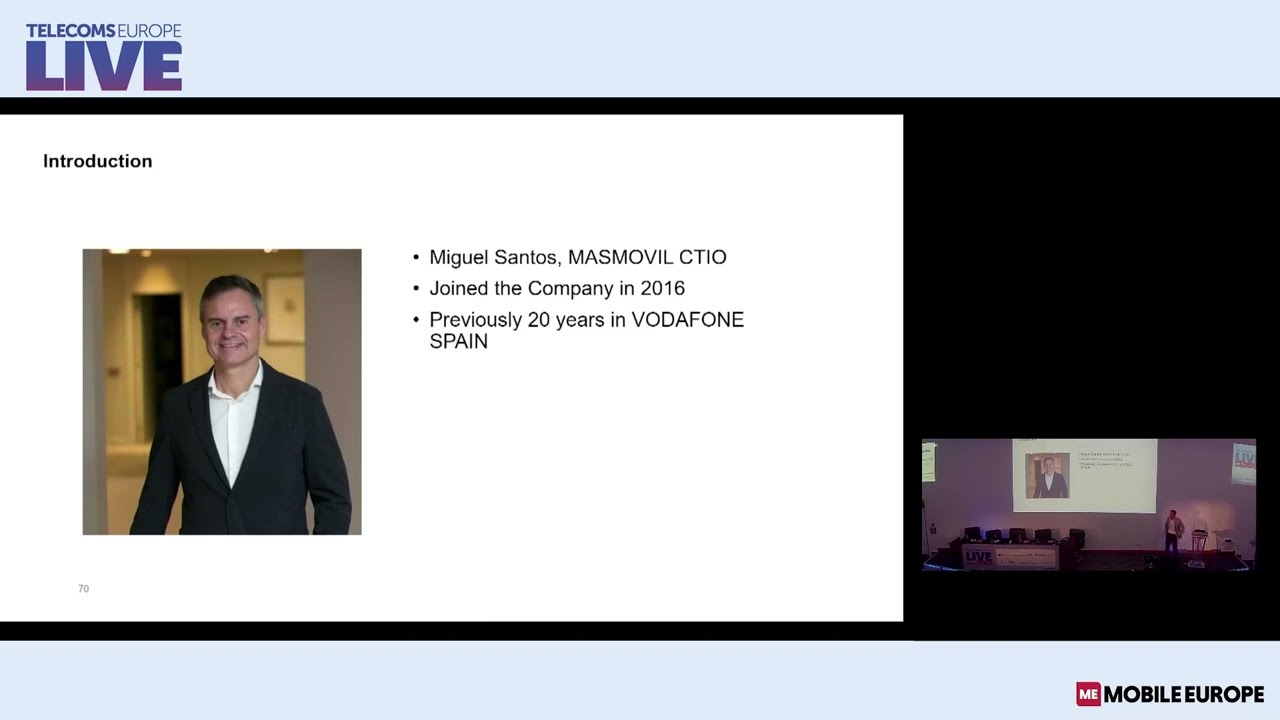The image is a slide from a PowerPoint presentation titled "Telecoms Europe Live" in blue letters at the top left corner, on a light blue background. It introduces Miguel Santos, labeled as the CTIO of Masmovil, displaying his photo on the left side. He appears to be around 45 years old, with dark hair graying at the sides, smiling and wearing a black suit with a white dress shirt. The slide details that he joined the company in 2016 and had previously spent 20 years at Vodafone in Spain. Below the introduction, there is text that says "ME" in a black box, followed by "Mobile Europe." To the right of Miguel’s image, there is a smaller image within the slide showing a man standing on a stage, possibly giving a presentation in front of a screen, with a purple-tinged wall in the background.